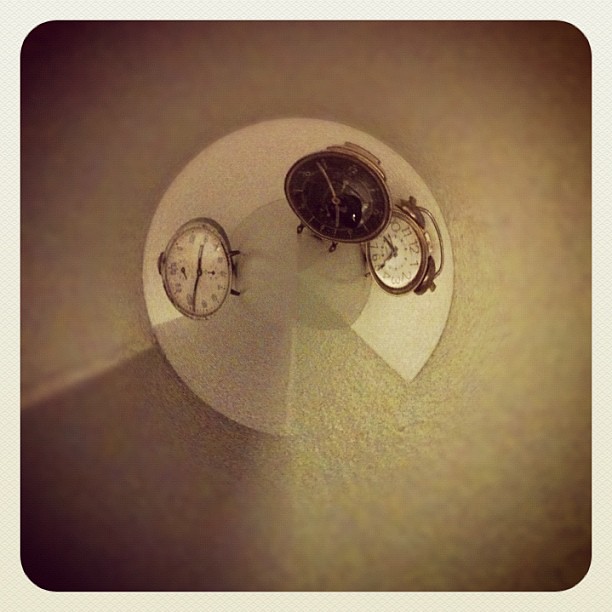The photograph features a collection of three retro, wind-up alarm clocks arranged on a unique background. Taken from an overhead perspective, the clocks are placed on what resembles a "Pac-Man" shape – a white circular form with a triangular wedge missing from the bottom. The image has a distinctive dark brown shade that gradually lightens toward the center, contributing to a vintage aesthetic. Each clock is distinct in design: one has a white face with metal parts and twin bells on top, displaying the time at 8:20. Another clock to its right has a black face, indicating approximately 6:52. The third clock, silver with a gray border, shows around 2:44 and is positioned on the left. The overall color palette is muted, featuring beiges, browns, and dark greens, enhanced by a yellowish filter that adds to the retro ambience. The image appears lower quality, with a fisheye effect and noticeable shadows, framed by a smooth, white border.